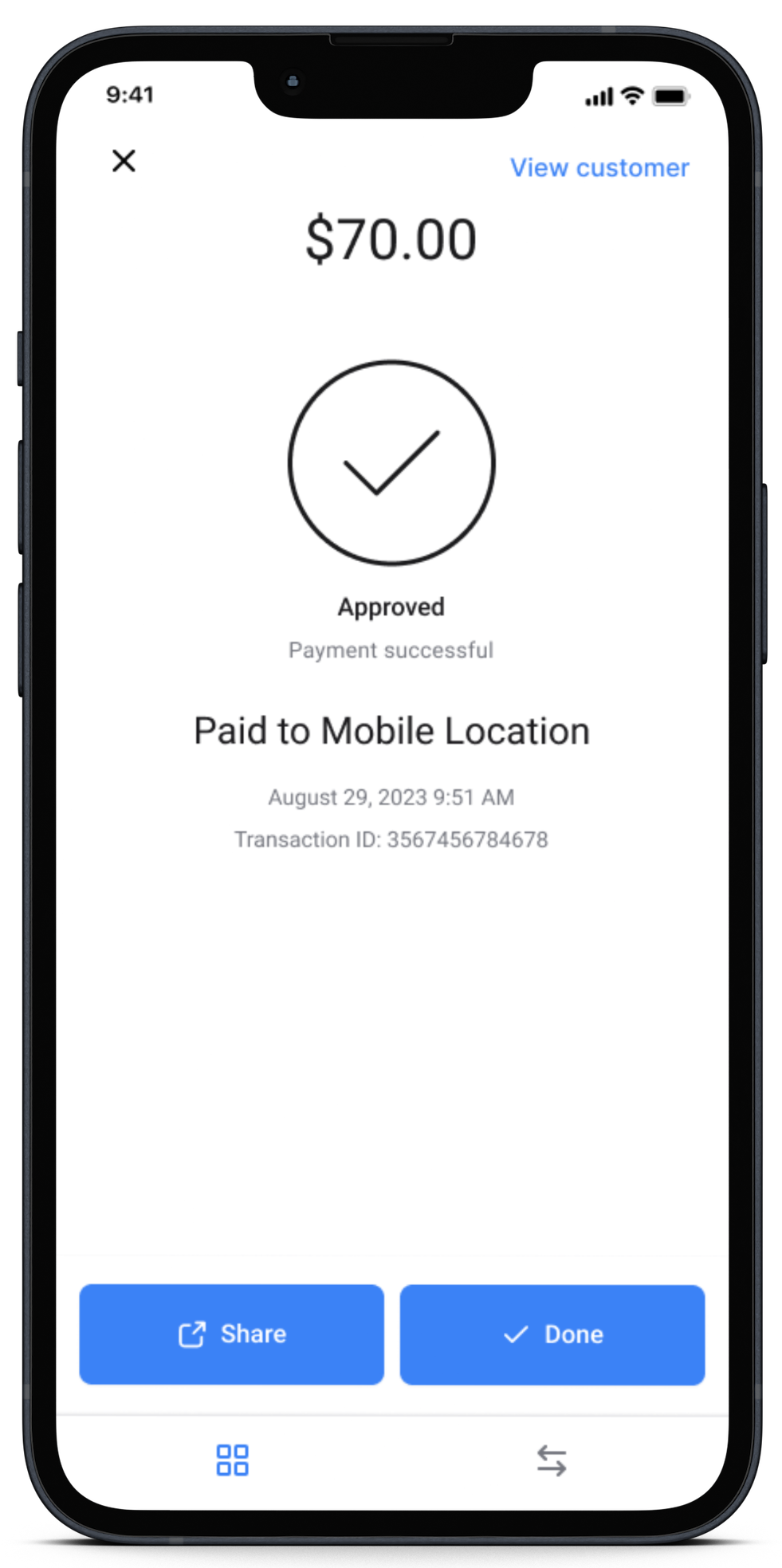**Detailed Caption:**

This image is a screenshot of a mobile application interface, likely tailored for business use, as indicated by the "View Customer" option in the top right corner. The interface displays a confirmation of a successful transaction, prominently featuring a green circle with a check mark and the message "Approved Payment Successful." The amount of $70 is displayed at the top, indicating the transaction value. Below, it specifies the payment details, stating "Paid to Mobile Location on August 29th, 2023, at 9:51 a.m.", followed by a transaction ID for reference.

At the bottom of the screen, there are two blue buttons labeled "Share" and "Done", allowing the user to either share the transaction details or mark the process as completed. The interface also highlights an active navigation icon in the bottom left corner, which consists of four squares arranged in a grid and is colored blue, suggesting it is the currently selected option. Additionally, there is another navigation icon in the bottom right corner, featuring two arrows pointing in opposite directions (left and right), but this icon is grayed out, indicating it is not currently active.

The layout and functionality of the app suggest it is designed for facilitating financial transactions on the go, potentially for a business managing customer payments.